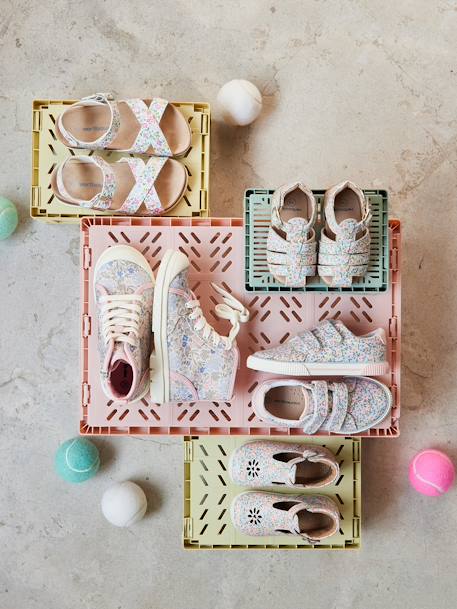Overhead color photograph showcasing an assortment of baby and child shoes arranged on a white marble background. The scene includes several plastic boxes in different colors: a yellow box at the top, a large pink box in the middle, and a smaller green box at the top right corner, with another yellow box at the bottom. 

At the top, there is a pair of child-sized sandals featuring an ankle strap and an X-shaped design over the toe area, adorned with a floral pattern. On the green box, there are two baby sandals with three straps across the toe area. On the left side of the pink box, a pair of high-top sneakers with white laces and a floral design are displayed, one lying on its side to showcase the pattern. 

At the bottom right corner of the pink box, a pair of slip-on sneakers with Velcro straps is visible. Positioned on the bottom box, a pair of baby shoes with an ankle strap and a buckle closure, featuring a perforated flower design on the toe area, can be seen. Scattered throughout the image are numerous multicolored tennis balls in shades of white, green, pink, and blue, adding a playful touch to the composition.